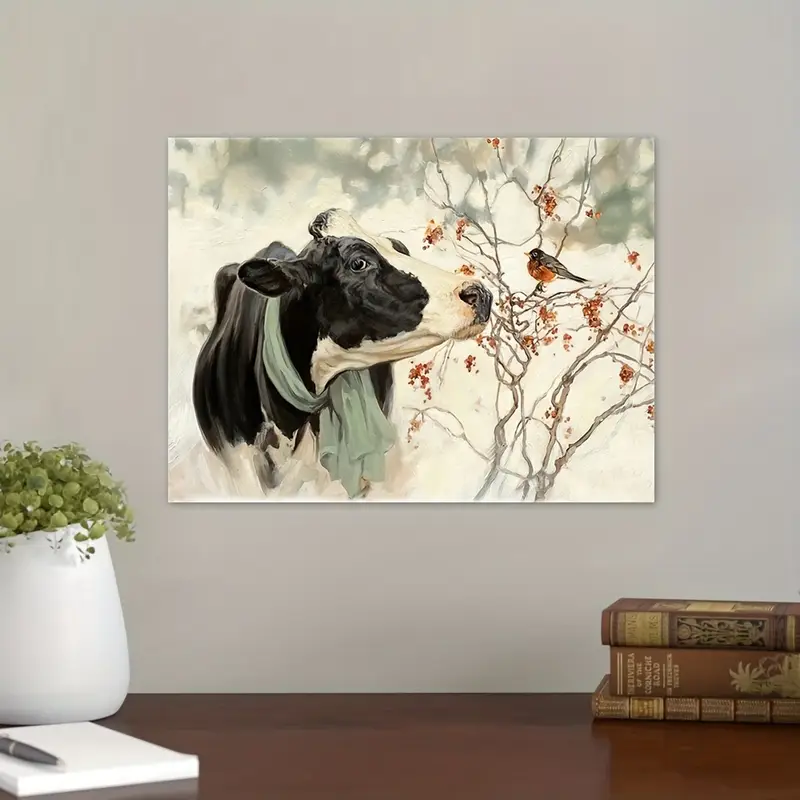The image displays a detailed and vibrant scene centered around a rectangular painting mounted on a whitish wall. The painting features a black and white cow with a blue scarf wrapped around its neck, looking to the right at a small red-bellied bird perched on a branch adorned with thin twigs and red berries, suggesting a winter setting. Below the painting is a dark brown wooden table. On the table's bottom left corner, there is a stack of three brown books of varying shades from dark to light. Adjacent to the books, there is a white vase with small green plant leaves extending from it. In front of the vase rests a white notebook with a black pen placed on top. The scene appears highly detailed, potentially computer-generated, capturing a cozy and rustic ambiance.